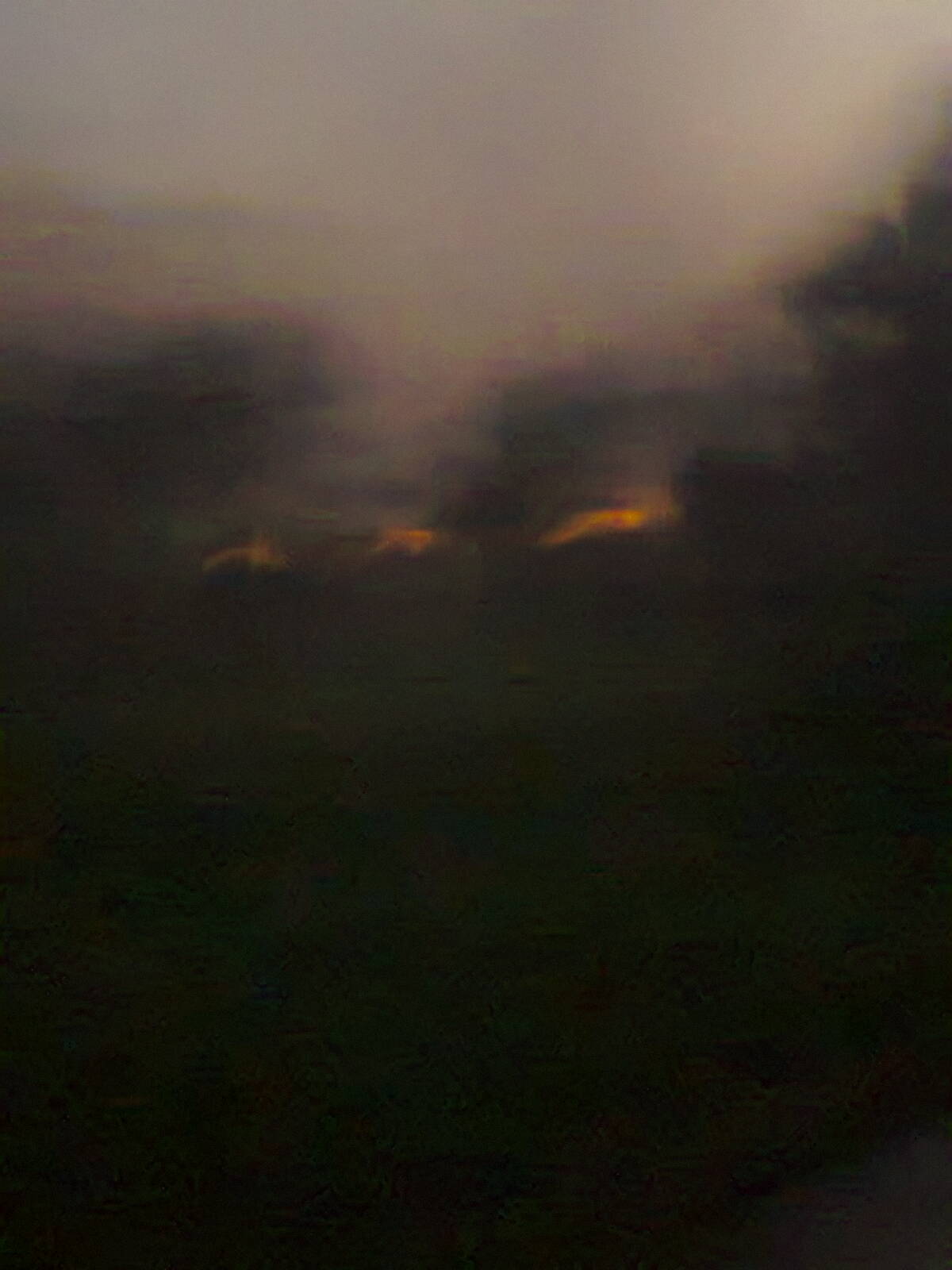This photograph, taken in portrait mode, reveals a dramatically blurry landscape dominated by dark, stormy clouds. The overwhelming darkness permeates the bottom half of the image. This area, nearly pitch black, obscures any detail that might lie within. Moving upward, the clouds transition from an impenetrable darkness to a lighter dark gray shade, adding a faint delineation. Centered within this gloom, three distinct sections of radiant orange punctuate the scene, appearing almost like curves of fire—possibly indicative of the sun either setting or rising and casting a brilliant glow on the clouds. The very top of the image shows a slightly clearer portion of the sky, marked by a less dense gray, suggesting the formation of storm clouds rolling in and covering what might otherwise be a clearer expanse. The blurry composition of the photograph leaves room for interpretation, hinting at possible elements such as mountains or trees outlined against the dimming sky, accentuated by the fiery hues amidst the bleak backdrop.